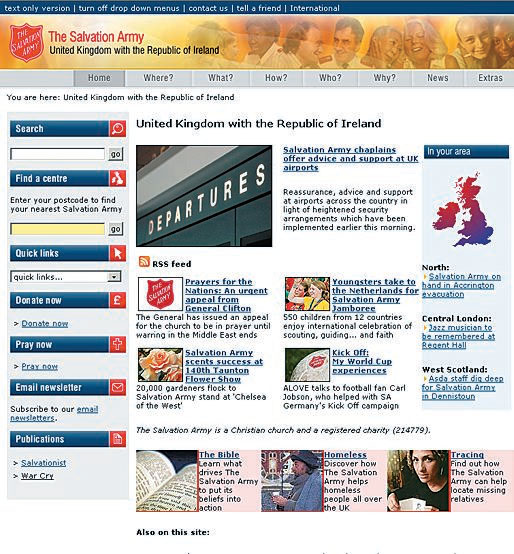This is a screen capture of the Salvation Army's website, prominently featuring a structured and user-friendly interface. At the very top, a blue taskbar displays links in white text for accessibility options, including "text-only version," "turn off drop-down menus," and quick access to "contact us," "tell a friend," and "international" sections.

Below the taskbar, a wide banner spans the top of the page, displaying a diverse group including doctors, nurses, elderly women, and children of different ethnic backgrounds, symbolizing the Salvation Army's inclusive mission. On the far left of this banner, the iconic red Salvation Army shield is accompanied by the organization's name in white text, "The Salvation Army." Adjacent to it, the text "The Salvation Army United Kingdom with the Republic of Ireland" stands out in red.

The website features a navigation menu with tabs labeled "Home," "Where," "What," "How," "Who," "Why," "News," and "Extras," facilitating easy access to various sections. Directly beneath this menu, the text confirms the user's location within the site: "You are here: United Kingdom with the Republic of Ireland."

Prominent on the page is an announcement detailing the support offered by Salvation Army chaplains at UK airports. The message highlights the reassurance, advice, and assistance provided in response to newly implemented heightened security measures. Additionally, the page features articles and resources such as "Prayers for the Nations" and an "Urgent Appeal from General Clifton."

The site also includes a section guiding users to find local centers, categorized by regions like North, Central London, and West Scotland. On the far left sidebar, there are functional search bars and quick links for "Search," "Find a Center," "Quick Links," "Donate Now," "Pray Now," "Email Newsletter," and "Publications."

Overall, the detailed layout and comprehensive resources reflect the Salvation Army's commitment to community support and accessibility.